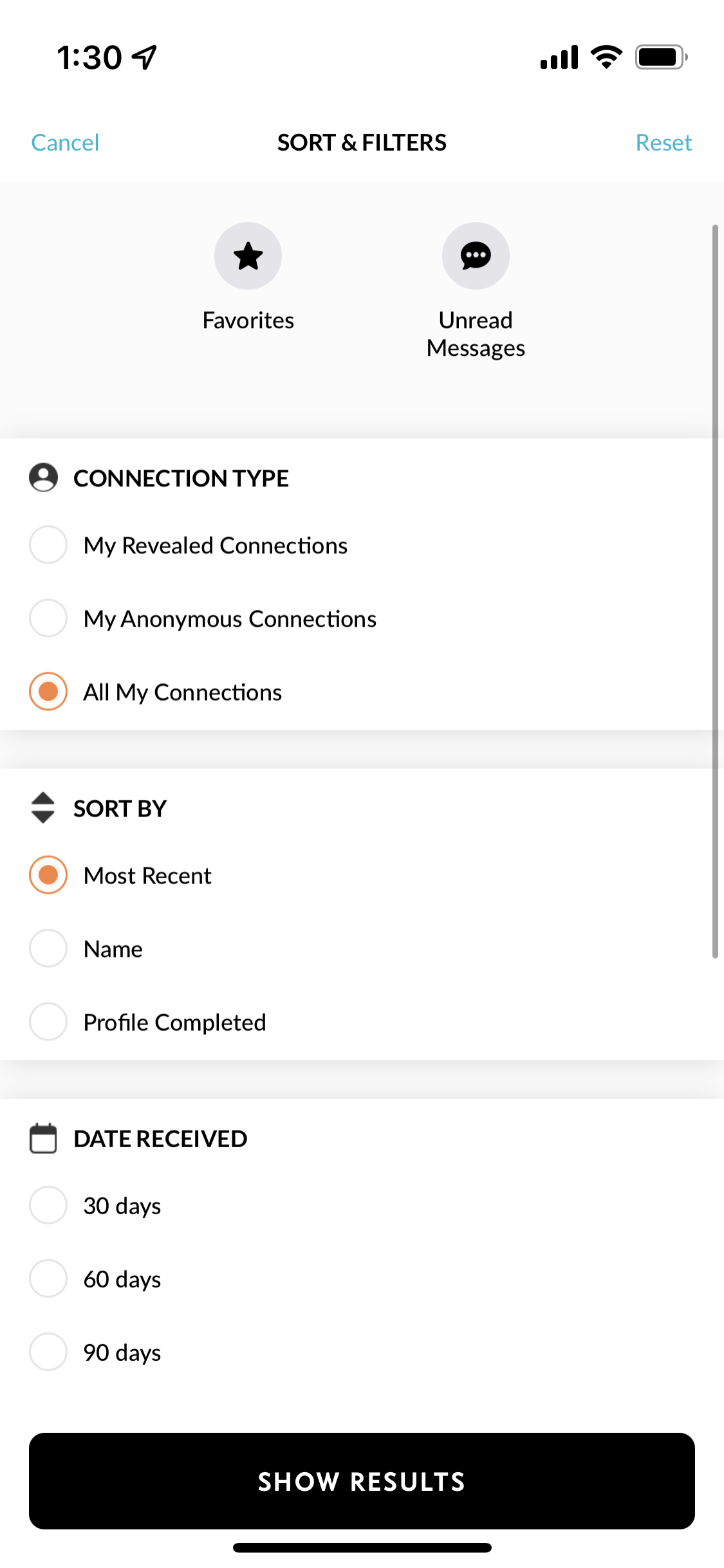The image displays a smartphone screen with a sorting and filtering interface for managing connections and messages. At the top, there is a navigation bar with a "Cancel" button on the left and a "Reset" button on the right. Below this, users can filter their connections and messages by selecting options such as "Favorites" or "Unread Messages."

A section labelled "Connection Type" offers multiple selections, including "All My Connections," "My Revealed," and "My Anonymous." Users can filter their connections based on these categories. The interface also includes a "Sort By" option where users can choose to sort their connections by "Most Recent," "Name," or "Profile Completed."

Another section, "Date Received," is available but not yet selected by the user. It offers options to filter connections by the dates received: "30 days," "60 days," or "90 days." At the bottom of the screen, there is a prominent black button with the text "Show Results" in white, allowing users to apply the selected filters.

Additional interface details include an indicator showing "130" on the top left corner and status icons for full signal bars, strong Wi-Fi, and a full battery in the top right corner. The overall background of the screen is white, and selecting options highlights them with an orange dot, indicating active filters. The interface appears user-friendly, enabling users to efficiently manage and sort their connections.